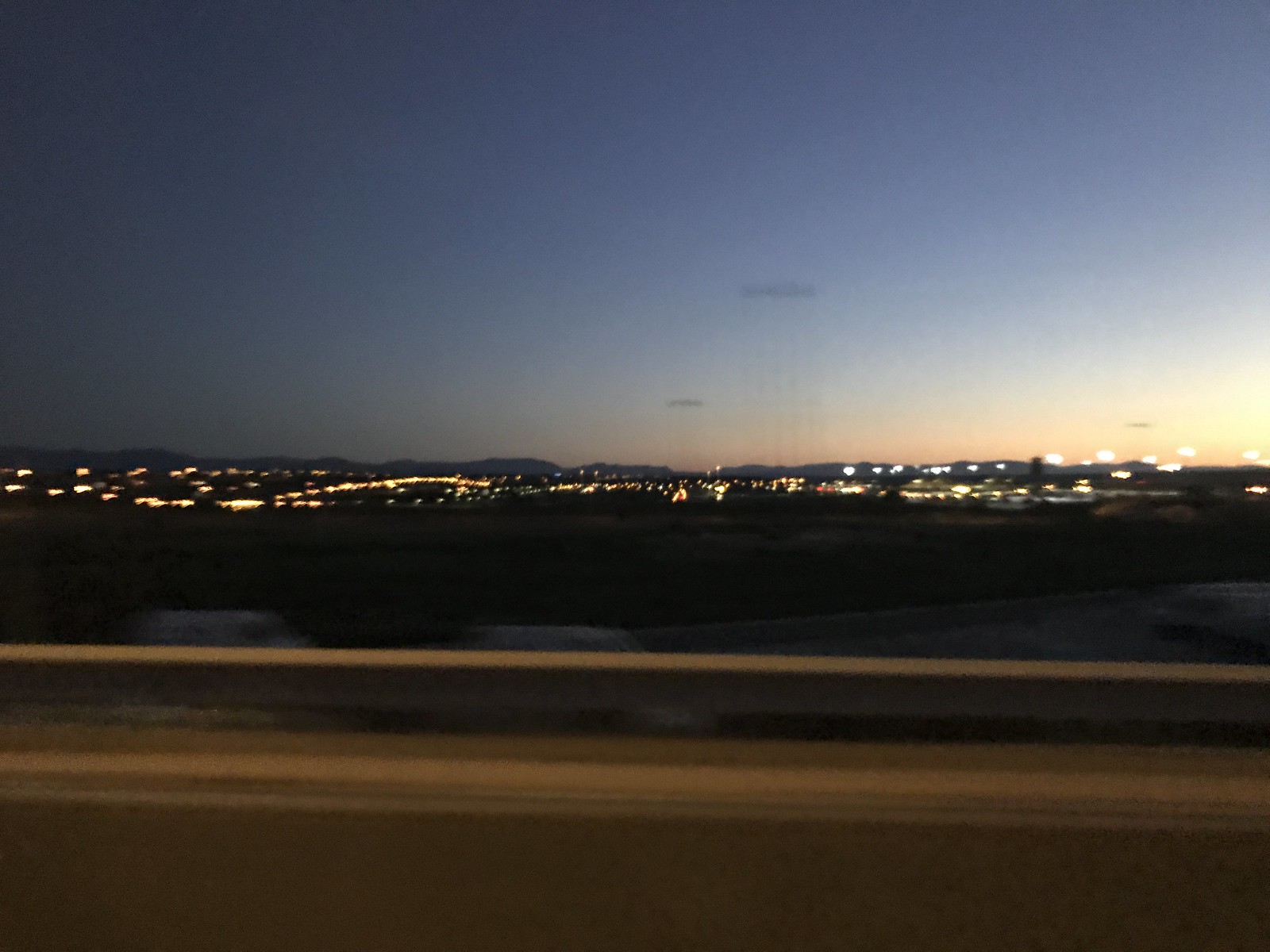This image captures a scenic view taken in motion from the passenger side of a moving car, likely on a highway or bridge. The foreground is slightly blurred, featuring a street and a highway-type barrier. Beyond the barrier, there is a dark, hilly terrain suggesting a deserty or less vegetated area. In the midground, a city or town stretches across the photo, its myriad lights twinkling vividly as the day transitions to night. The sky, a gradient from dark blue in the upper left to a softer pinkish hue toward the middle and right, indicates an impending sunset, primarily illuminating the right side of the image. In the backdrop, the silhouette of irregular mountains or hills frames the well-lit cityscape, enhancing the picturesque twilight scene.